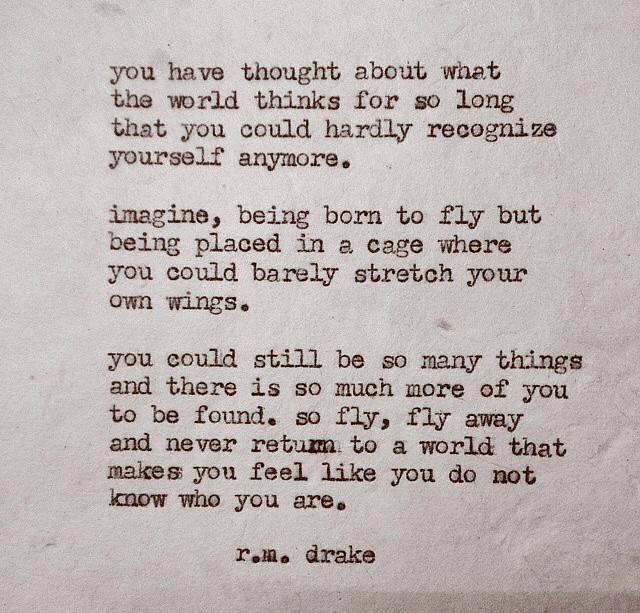The square image features a poem or prose, typewritten in lowercase on a slightly crinkled and grainy off-white paper resembling old fiber paper. The typewriter font is a burgundy to almost black hue. The text reads: "you have thought about what the world thinks for so long that you could hardly recognize yourself anymore. imagine, being born to fly, but being placed in a cage where you could barely stretch your own wings. you could still be so many things, and there is so much more of you to be found. so fly, fly away and never return to a world that makes you feel like you do not know who you are." The piece is attributed to R. M. Drake.